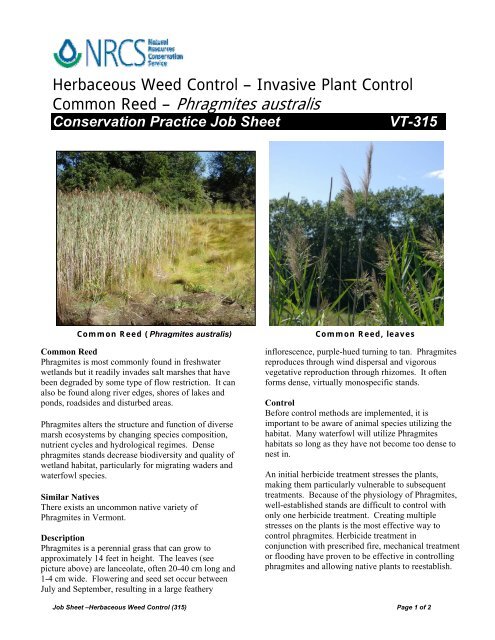The image is a detailed informational sheet or poster about the herbaceous weed control of invasive plant species, specifically the common reed (Phragmites australis). At the top, it prominently features the blue logo of the Natural Resources Conservation Service (NRCS), which looks like a teardrop seated in a rocking chair. Alongside the logo, in blue capital letters, is "NRCS," which stands for Natural Resources Conservation Service. Below this, in black letters, it reads "herbaceous weed control, invasive plant control, common reed, Phragmites australis."

To the side, there is a black stripe with white text that states, "conservation practice job sheet." Adjacent to this, it is labeled "BP-35." Below these texts, there are two images showcasing the common reed. The left picture features a field overrun with weeds against a backdrop of green trees, while the right image, set among the same green trees, shows leaves resembling those of corn stalks, though they are not corn.

Additional textual information follows, including several paragraphs describing the common reed's habitat, including freshwater wetlands, salt marshes, river edges, lakeshores, roadsides, and disturbed areas. The text highlights the impact of Phragmites on marsh ecosystems, noting its alteration of species composition, nutrient cycles, and hydrological regimes, as well as its negative effects on biodiversity and wetland habitats, particularly for migrating waders and waterfowl species. It also mentions a similar, less common native variety of Phragmites in Vermont. Overall, the document serves as a comprehensive resource on weed management practices for Phragmites australis.